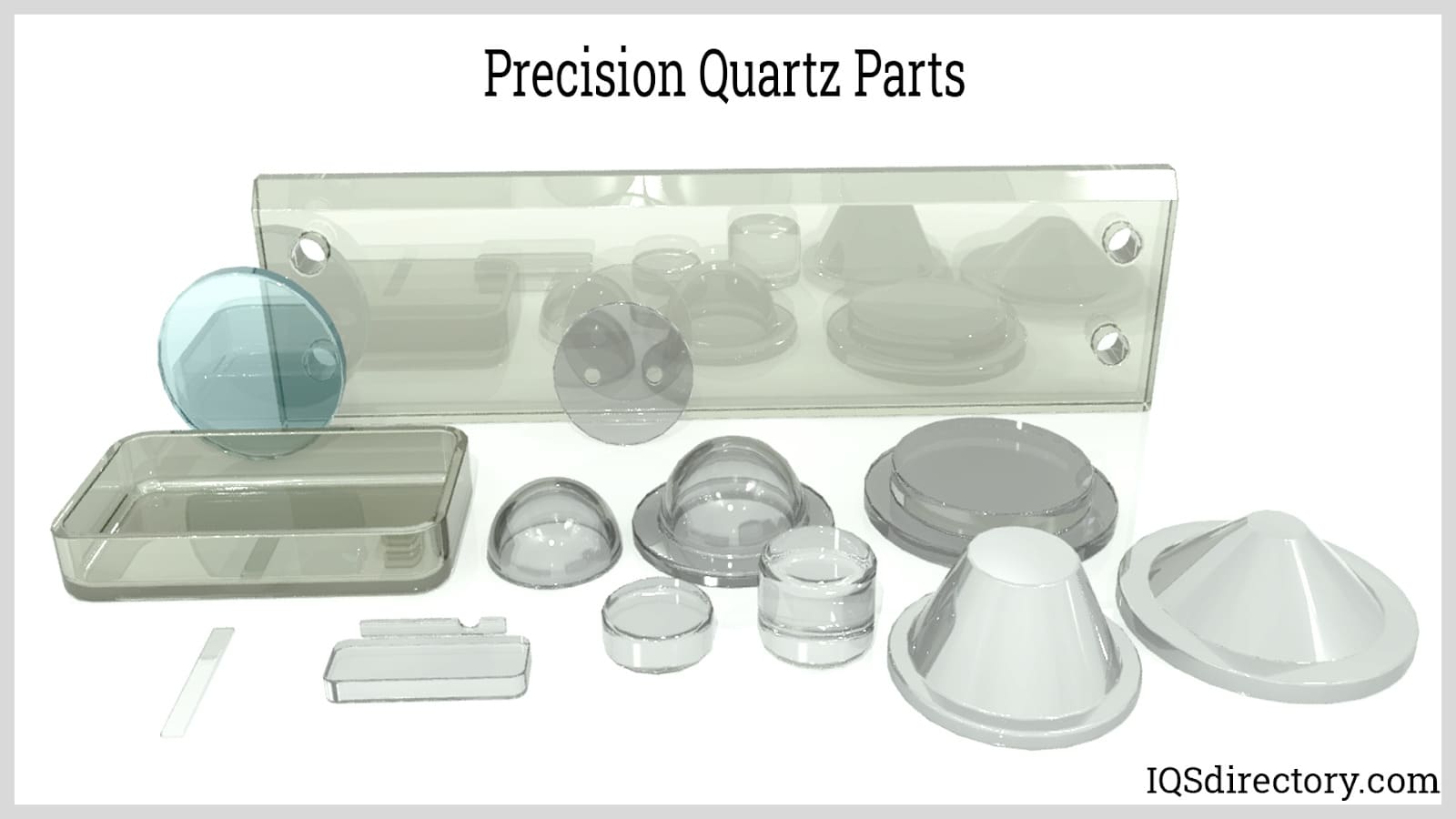The image is a detailed graphic showcasing various precision quartz parts against a white background, bordered by a light gray rectangular frame. At the top center, in black font, it reads "Precision Quartz Parts." Several geometrically-shaped quartz parts, which are mostly spherical, conical, flat, circular, and rectangular, are displayed in the middle of the image. The parts range in color from gray, white, to bluish, and have a transparent or translucent quality. 

Notable components include:
- A large, transparent rectangular piece with a reflective surface and four drilled holes, two on each side.
- Small round plates, including a completely transparent blue one.
- Cone-shaped caps, some with flat cones and others with pointy cones.
- Dome-shaped pieces that resemble caps.
- A rectangular ashtray-like structure made of darker quartz.
- Upside-down, bubble-shaped pieces and rounded cylinders, including one with a dome and another resembling a flat bowl.
- Small and taller round containers, and bowls turned upside down in white and gray quartz.

In the bottom right corner, "iqsdirectory.com" is written in black font, completing the professional presentation of the quartz components.